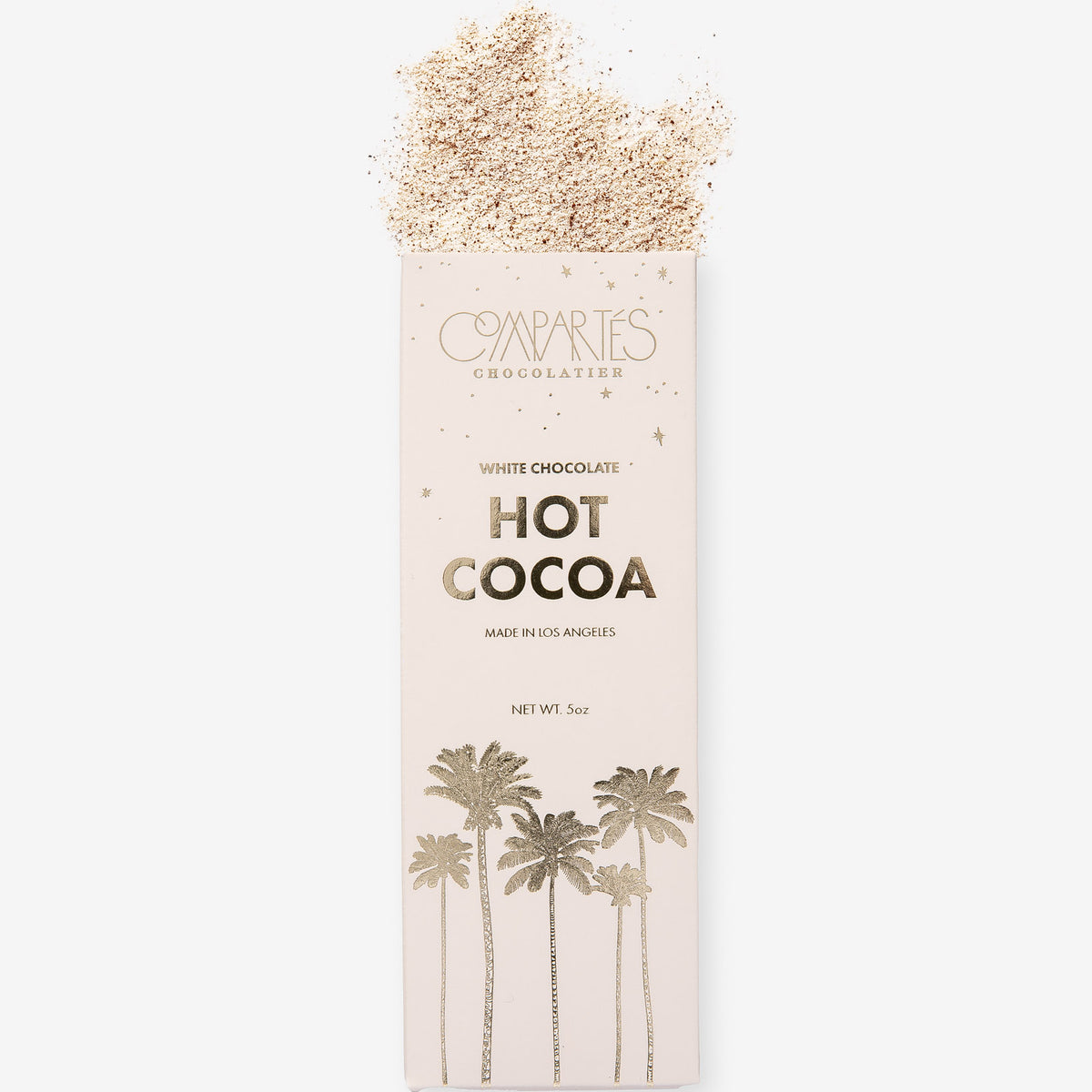This image depicts a tall, narrow, rectangular package of Compartes Chocolatier White Chocolate Hot Cocoa, made in Los Angeles, with a net weight of 5 ounces. The packaging is predominantly black and white with a very faded pink hue, giving it a sleek, minimalistic appearance. At the top of the package, there is white chocolate hot cocoa powder spilling out onto a white surface, with visible crumbly and powdered bits. The middle section prominently features the Compartes Chocolatier branding with an accent on the "E." The bottom part of the package showcases an illustration of five tall and thin palm trees, reminiscent of those commonly seen in Los Angeles. The light source in the image comes from the left, casting a subtle shadow on the right side of the package.